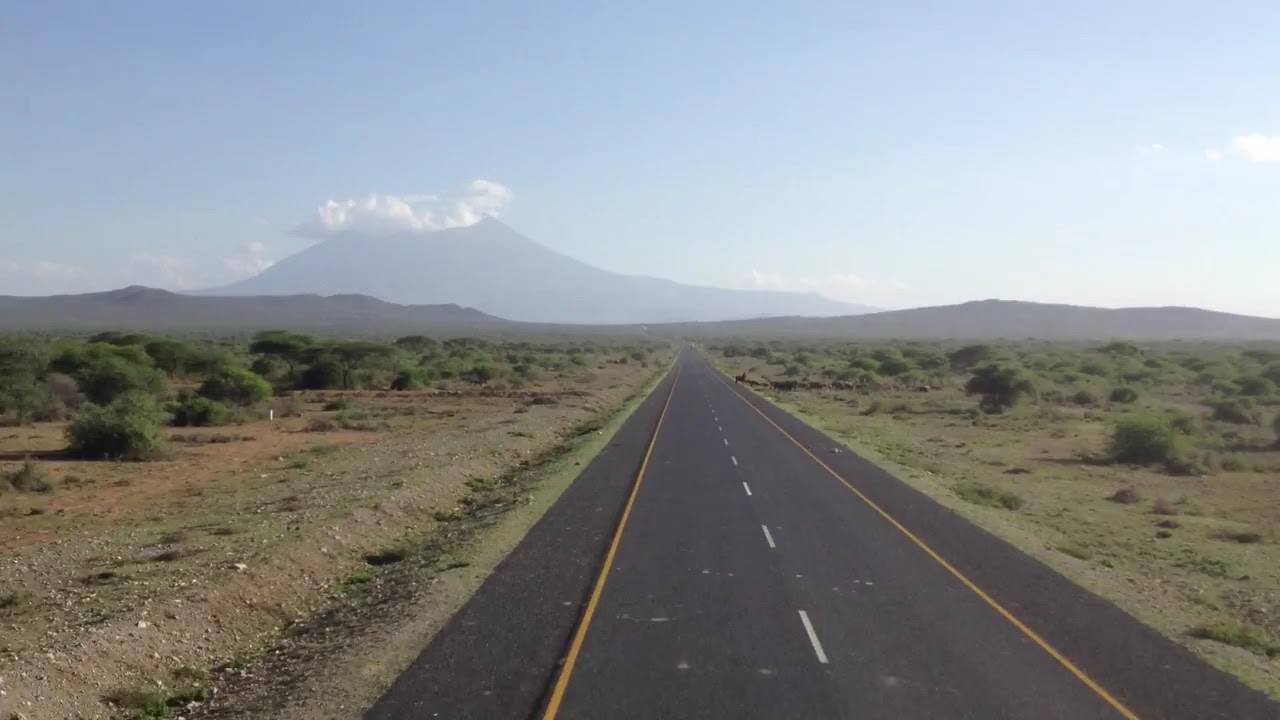The image depicts a long stretch of a two-lane highway that begins near the center of the frame and extends out to the right-hand side. The road is paved with dark tarmac and features solid yellow lines on the edges and a dashed white line running down the middle. The landscape on either side of the road is primarily flat, dotted with dry-looking bushes and patches of grass, evoking a semi-arid or desert-like environment. To the left of the road, a ditch runs parallel to the pavement. In the distance, the terrain transitions to rolling hills and eventually a large, muted mountain that dominates the background, surrounded by a few scattered clouds. The sky is predominantly clear with a hint of haze, possibly suggesting a recent nearby fire or simply the natural atmospheric conditions of the region. The image is devoid of any visible occupants or vehicles, enhancing the sense of rural solitude. The scene is captured during the daytime, under a bright but slightly hazy sky, adding to the overall tranquil and isolated mood of the landscape.